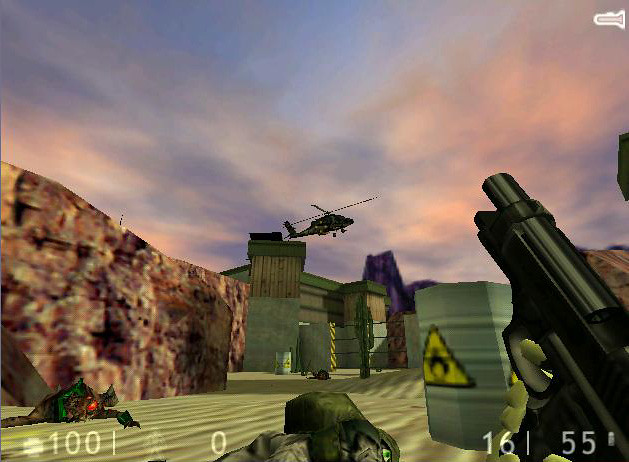In this vivid scene from an older first-person shooter video game, the sky is painted in hues of pink, purple, and blue, indicating that the sun has set. Dominating the skyline is a green military helicopter, appearing to take off above a large gray, beige, and green bunker or military building. Toward the left of the image, a brick stone wall is partially visible, near which lies the body of a character who has been hit by gunfire. The foreground is filled with various elements of environmental storytelling. There are several barrels scattered around, likely marked with caution signs for nuclear waste, sporting a yellow triangle with a black center. Among them, one green barrel and another silver container display these toxic chemical warnings. The interface at the bottom of the screen reveals crucial gameplay information: a score of 100, which signifies health points with a cross-shaped logo, alongside a vertical white line pointing next to an outline of a character and a white zero indicating the player is down to the last life. To the right, a massive black gun, held by the player, is pointed forward, likely aimed at the helicopter. The ground level showcases a diverse terrain with low cliffs and what might be dead monsters or bugs in green, lying next to rocks. The intricate details of this graphics-laden scene capture the essence of a classic, tactical combat scenario, blending elements of danger and strategy against the dramatic backdrop of a colorful twilight sky.